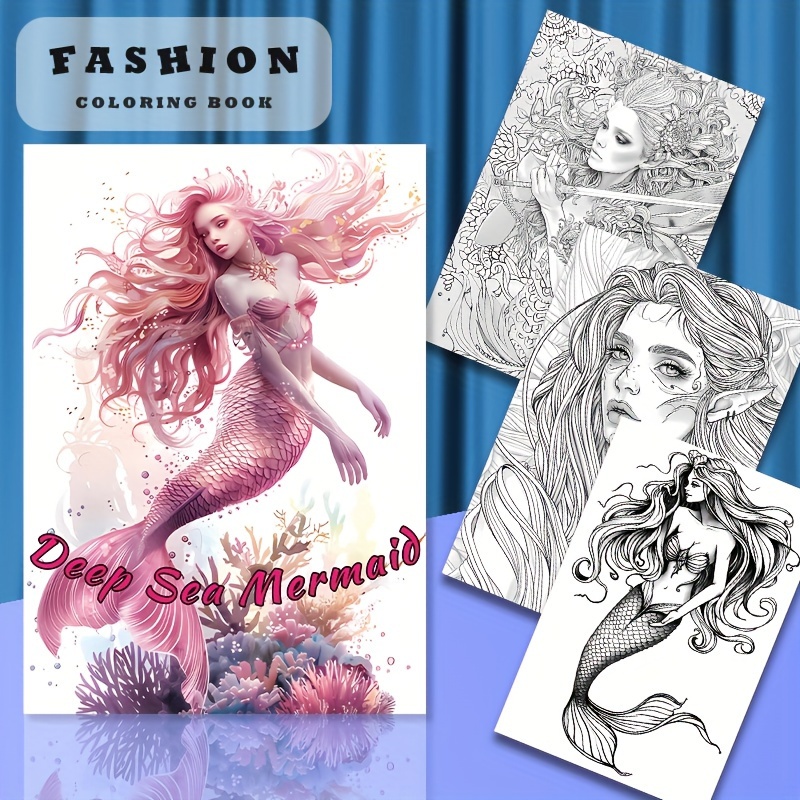The image is a photograph of illustrations centered around a mermaid theme, presented as an advertisement for a fashion coloring book titled "Deep Sea Mermaid." On the left side, there's a prominent rectangular illustration featuring a pink and golden mermaid with long, rose-gold hair and a detailed fishtail, positioned against a white background. Above this image, the words "Fashion Coloring Book" are inscribed in the top left corner. To the right, three black-and-white sketches of elegant, non-human women—mermaids or possibly elves, suggested by their features—are displayed, ready to be colored. These illustrations are laid out on a table draped in blue, framed by a matching blue curtain in the background. The pink mermaid in the main illustration also wears a pink seashell bra, enhancing her ethereal beauty. This composition, likely computer-generated, emphasizes a stylish, fantasy-driven aesthetic designed to appeal to creative coloring enthusiasts.